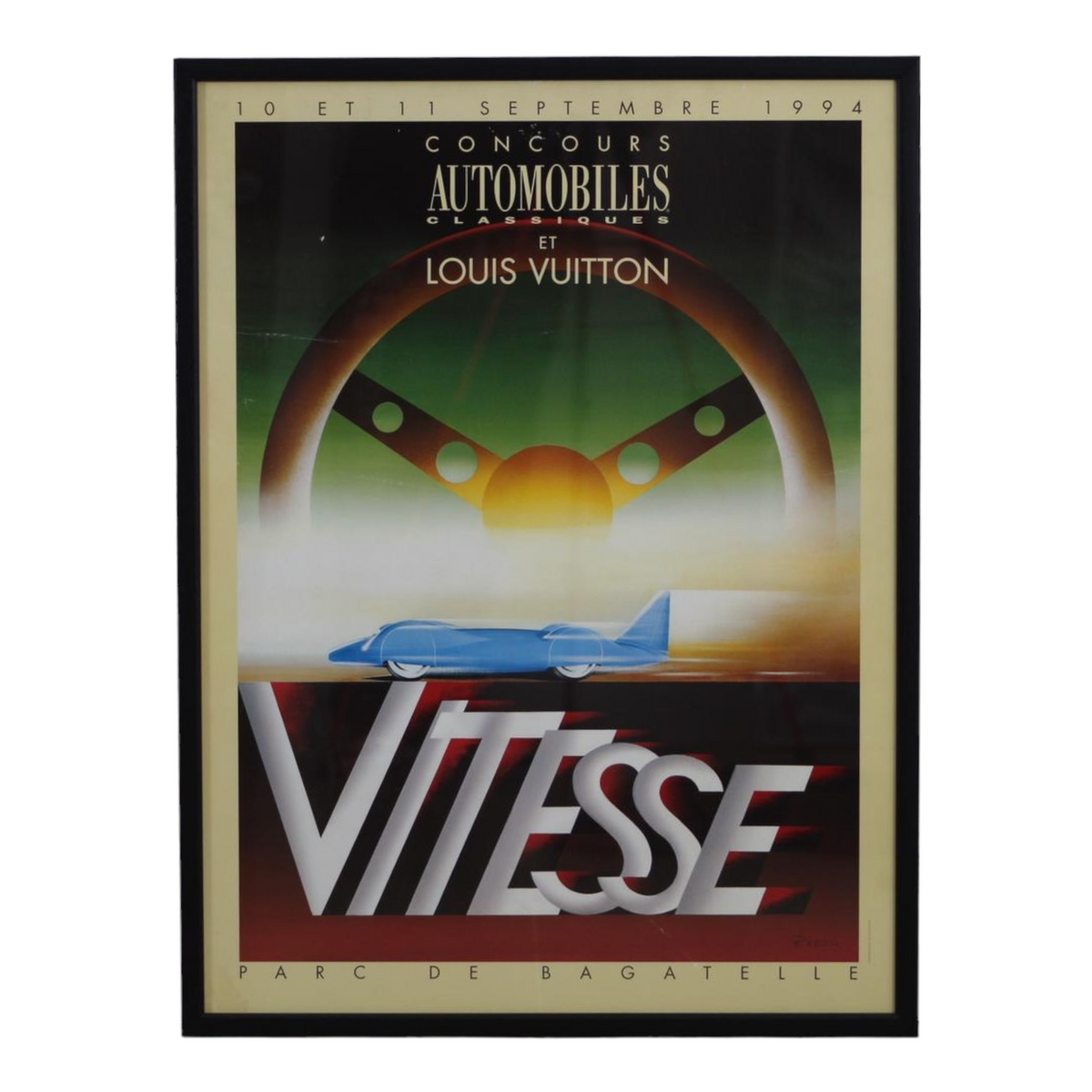The image depicts a framed vintage poster, predominantly featuring a sleek, blue car with a design reminiscent of an airplane, complete with a long body, aerodynamically enshrouded wheels, and a cockpit-like front. The car is shown racing from the left side of the frame, producing white speed streaks. Above the car, there's an illustration of a distinctive steering wheel with a Y-pattern and circular cutouts. The top portion of the poster, set against a beige background, announces "10th and 11th September, 1994" and additional text in French, including "Parc de Bagatelle" and "Concours Automobiles Classique et Louis Vuitton." Below the car, on a vibrant red background, the word "Vitesse" is prominently displayed in bold white letters, indicating speed in French. The color scheme of the poster transitions from black at the top to green and then to a whitish-yellow, finishing with red and black at the bottom. The entire poster is framed in black, set against a white background.